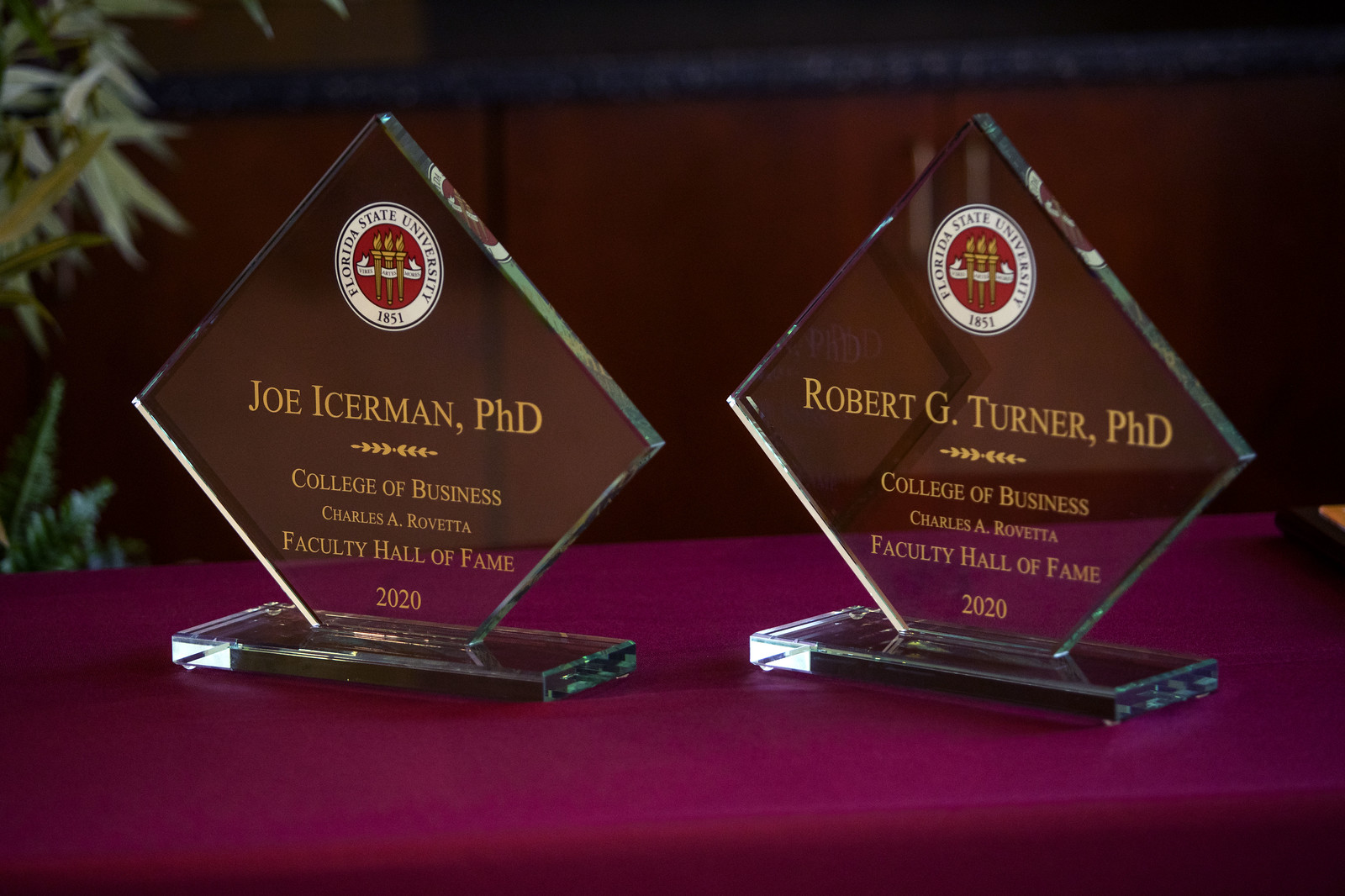The image showcases two elegant, transparent diamond-shaped awards set atop a square base, perched on a table draped with a crimson, velvety tablecloth. The awards, reflecting a glass-like clarity, are almost identical except for the inscriptions. Both awards honor esteemed members of the Florida State University's College of Business, recently inducted into the Charles A. Rovetta Faculty Hall of Fame in 2020. The left award is inscribed with "Joe Iserman, Ph.D." and the right with "Robert G. Turner, Ph.D.," both in gold lettering. Above the inscriptions, each award features the Florida State University emblem, which includes a circular white background encircling a smaller red circle that houses three orange torches intertwined with a white ribbon. The emblem also notes the university's founding year, 1851. In the backdrop, there is a brown wall with blurred cabinet handles visible near the center, and to the left, an indoor ficus tree adds a touch of greenery to the setting.